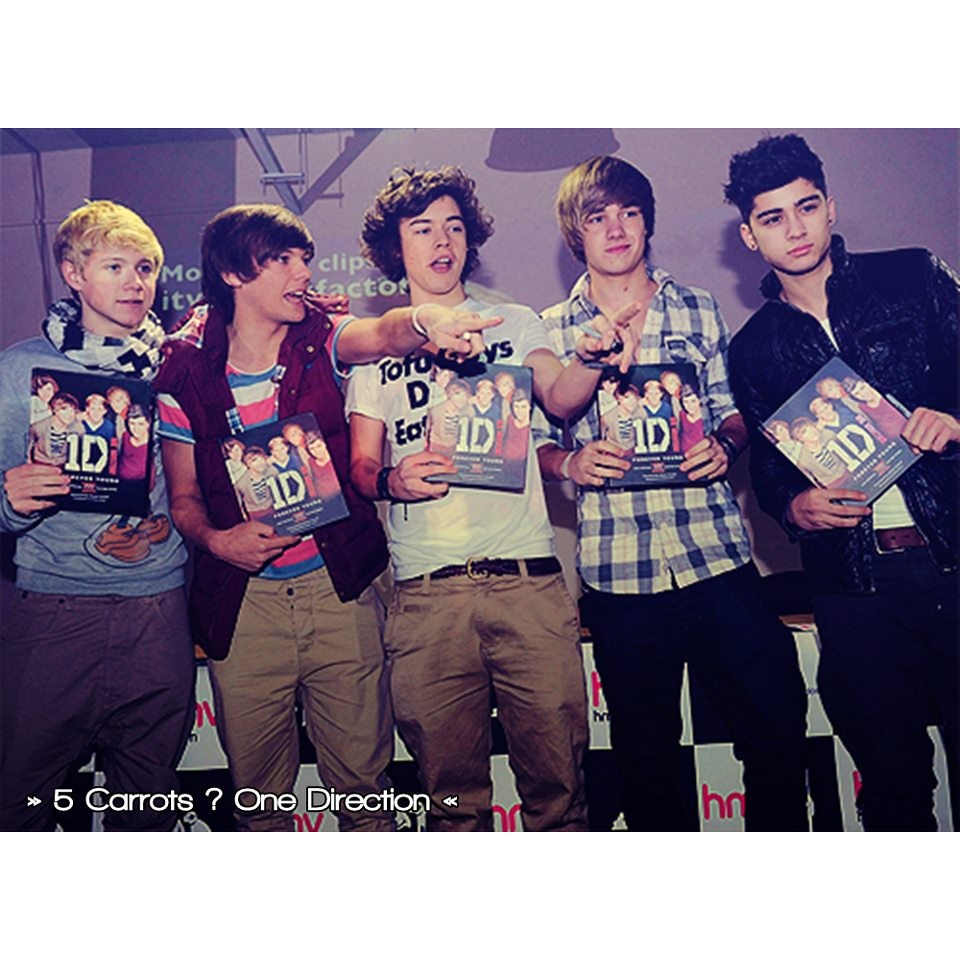This color photograph captures the British-Irish boy band One Direction in their early years, likely when they were around 16 to 18 years old. The five young men are standing side by side against a light purplish background with some darker shadows and white lettering that partially reads "five carats One Direction" and some other words including "clips" and "factor." Each member is holding up a CD or book displaying their image with a prominent white "1D" on the cover. The band members are dressed in varied styles: two are wearing khaki pants while the other three have on darker-colored pants. Their shirts also differ; some are in t-shirts, others in long sleeves. Notably, the boy to the left has blonde hair and a scarf, while the member next to him with darker brown hair wears a vest over a striped shirt and khakis. In the middle, a young Harry Styles is easily recognizable in a t-shirt and khakis, pointing forward with one hand. The second-to-last boy sports a plaid shirt, and the final young man, with his dark hair styled up, completes the lineup, all holding the same "1D" picture.